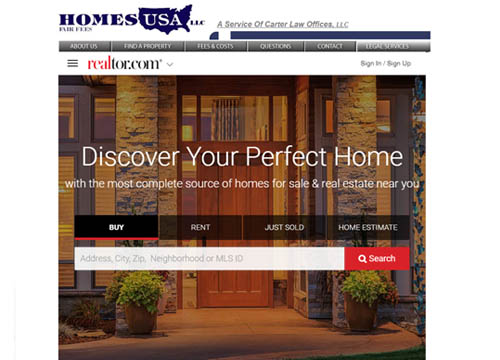The screenshot depicts the homepage of a real estate search platform integrated with a law office's website. In the top-left corner, the website is branded with "Homes USA LLC" in blue text featuring a motif of the United States, while the top-right corner labels it as "a service of Carter Law Offices LLC". Spread across the gray menu bar, options include "About Us," "Find a Property," "File Fees and Costs," "Questions," "Connect," and "Legal Services," each presented in white text.

Below the menu bar, several elements are arranged: a hamburger menu icon, the realtor.com logo with a drop-down menu option, and a "Sign In/Sign Up" link positioned to the far right. The main background image showcases a charming home at nighttime, featuring brickwork, plants, a wooden door, and numerous windows, though the interior details are indistinct.

Superimposed on this background are the words "Discover your perfect home with the most complete source of homes for sale and real estate near you" in white text. Beneath this tagline, a black bar with white text provides quick access options labeled "Buy," "Rent," "Just Sold," and "Home Estimate."

At the bottom of the image, a prominent search bar invites users to enter an address, city, zip code, neighborhood, or MLS ID. The search functionality is highlighted with a red search button bearing a white search icon.